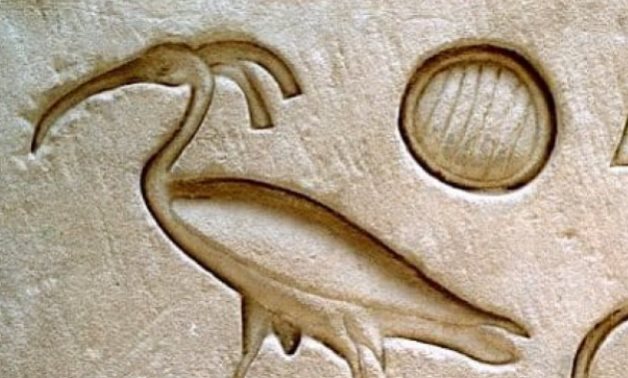The image depicts a detailed stone carving of a bird resembling a crane or ibis, intricately inscribed into a light brown, sandstone-like rectangle. The carving is roughly four to five inches wide and two to three inches high. The bird, oriented to the left, showcases a long, thin, and slightly curved beak, with a small, oblong-circular head and an extended neck. Two prominent feathers extend from the back of its head, flowing rightward then downward. The bird's body, long and narrow, tapers into legs that extend off the image's bottom. In the upper right corner, there's a carved circle with diagonal lines running through it. The background texture of the stone appears grayish with darker shading in between, suggesting a weathered and ancient look, possibly hinting at an Egyptian hieroglyphic origin. The surface beneath the bird and circle has a slightly raised, powdery white texture, adding depth to the carving.